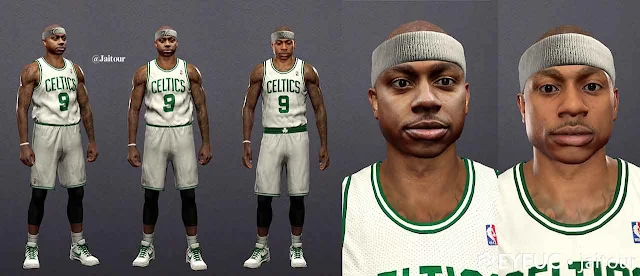This image features an African American basketball player dressed in a Boston Celtics uniform, specifically with the number nine. The composition on the left side of the image portrays three full-body views of the player in different stances: a slight side turn, a front-facing position, and another varied angle. Each of these poses showcases his white Celtics jersey with green accents, paired with matching white tennis shoes accentuated by green laces. 

To the right, the image highlights two close-up views of his face, both featuring a gray headband. This close-up captures the details of his facial expressions more clearly. 

Given the uniformity of the poses and the consistent facial features, it appears likely that this content is AI-generated. The color scheme throughout the image is predominantly gray, white, and green.